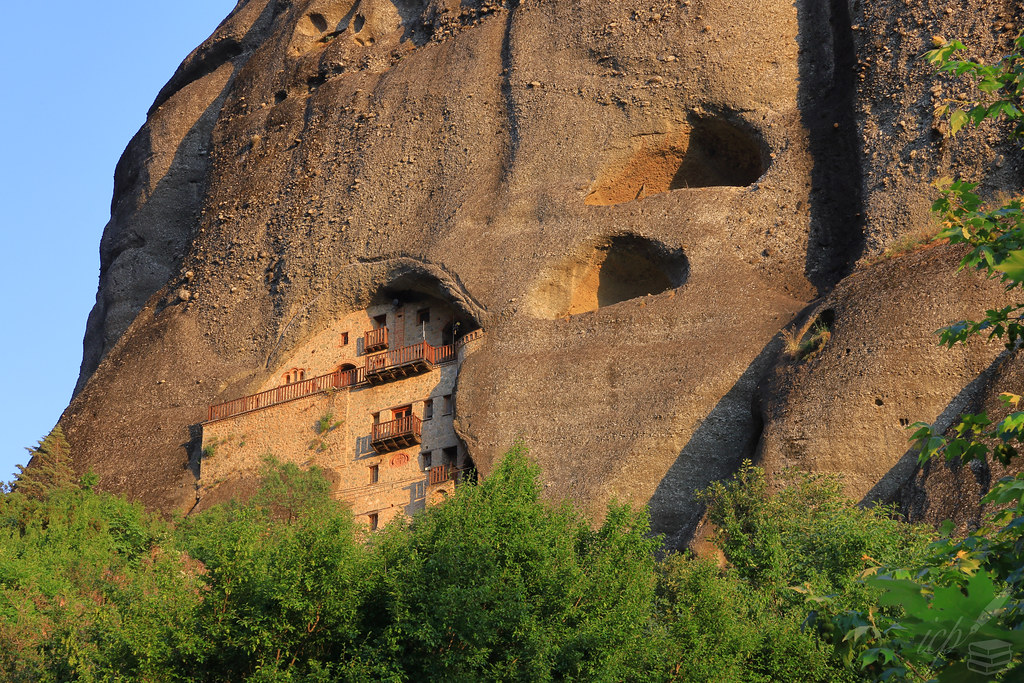The image features a grand rocky dome or mountainous formation with a beige-colored building intricately carved around the left side of the rock. This building, appearing extraordinary and unique, has square-cut windows and walk-out doors or balconies, each enclosed with reddish metal fencing. The structure, seemingly embedded into the rock, gives the impression of a seamless fusion with the natural formation. The dome itself is marked by various divots and cavities, with three major openings, one of which houses the building. The rock formation, with its bulbous protrusions, extends beyond the frame, standing against a backdrop of lush green trees and foliage that climb up from the bottom, mingling with the natural texture of the hill.